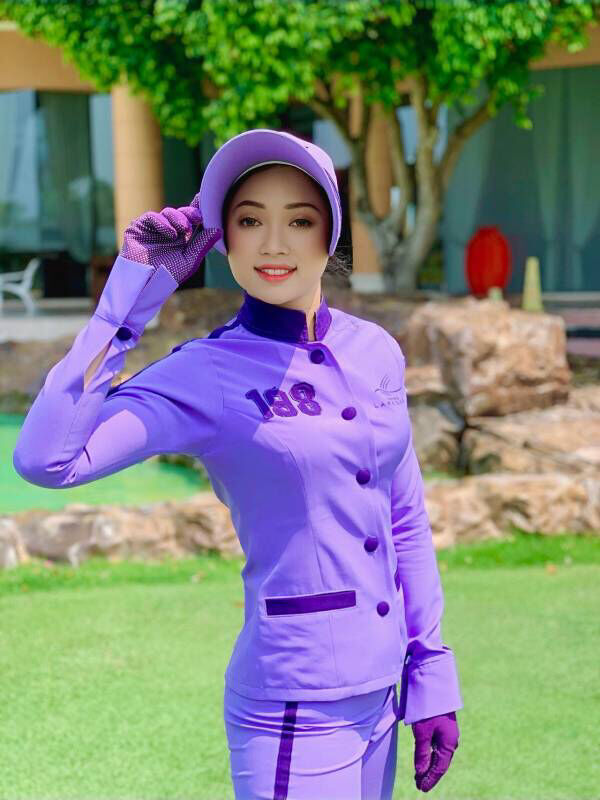This is a color photograph of a woman posing on a green lawn, likely in the front or back yard of a house. She is dressed in a distinct suit with a consistent tone of purple, comprising a jacket, pants, gloves, and a hat. The suit features blue highlights, including stripes on the sides of the pants and pockets, blue buttons, a blue collar, and the number "198" displayed on her right breast, alongside a bird logo. The woman is smiling and leaning slightly to her right, holding the brim of her matching purple hat with her right hand. She is adorned with red lipstick, eyeliner, and additional makeup. The lawn is bordered by a low stone wall with a higher stone wall behind it, and in the background, there is a tree, white lawn furniture, and what appears to be a blue building or patio with blue windows and a column.